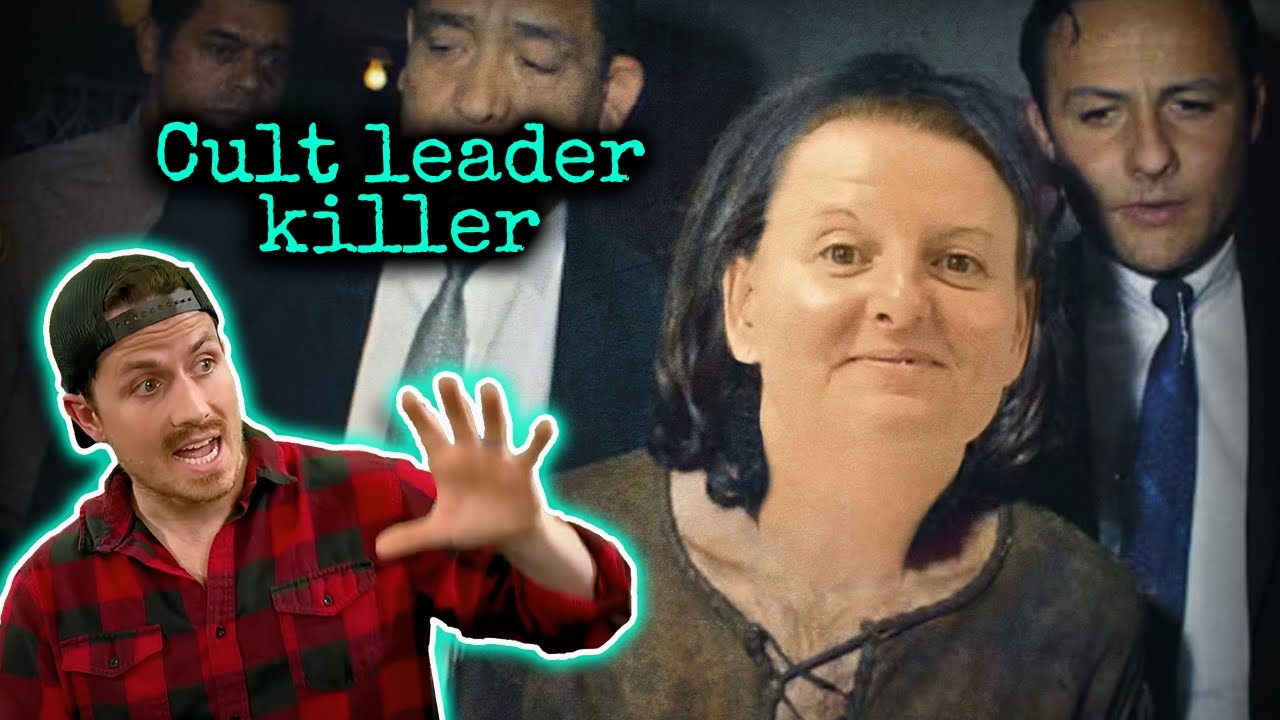The image appears to be a screenshot from a social media post. In the left corner, there is a superimposed figure of a man wearing a white baseball cap turned backwards. He has collarbone-length, short black hair and a mustache, with his lips pursed in a surprised expression. He is dressed in a blue and black checkered long-sleeve shirt and has a neon green outline around his body.

The main background of the image resembles a Ouija board, complete with candles positioned at the top and a central circle containing a star. A large red arrow dominates the picture, pointing towards a person’s head. This individual has eyes heavily rimmed in black; their left eye is entirely black, while the right eye appears gray with a white light in the center. The person’s mouth is slightly open, revealing missing teeth and forming a subtle, eerie smile. The figure also seems to be bald. The red arrow specifically highlights the left black eye, adding an unsettling focus to the image.